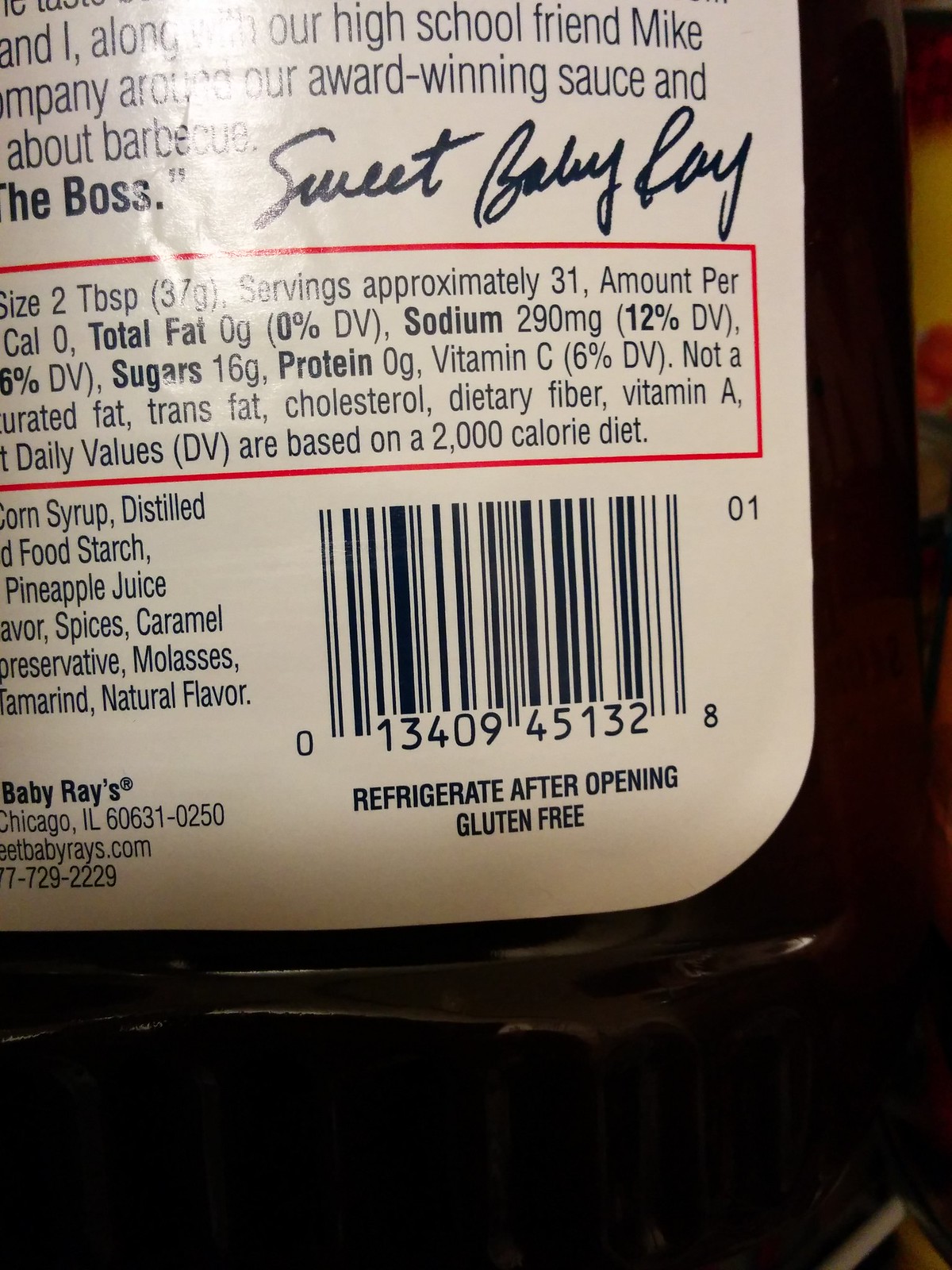The image features the back of a bottle of Sweet Baby Ray's barbecue sauce. The brand name, "Sweet Baby Ray's," is prominently displayed in a blue cursive font, resembling a signature, against the bottle's white surface. Although the nutritional information, ingredient list, and additional product details are partially obscured, the barcode is clearly visible and reads "01340945132." Below the barcode, the label indicates important storage and dietary information: "Refrigerate after opening" and "Gluten Free." The bottle itself is filled with rich, brown barbecue sauce.